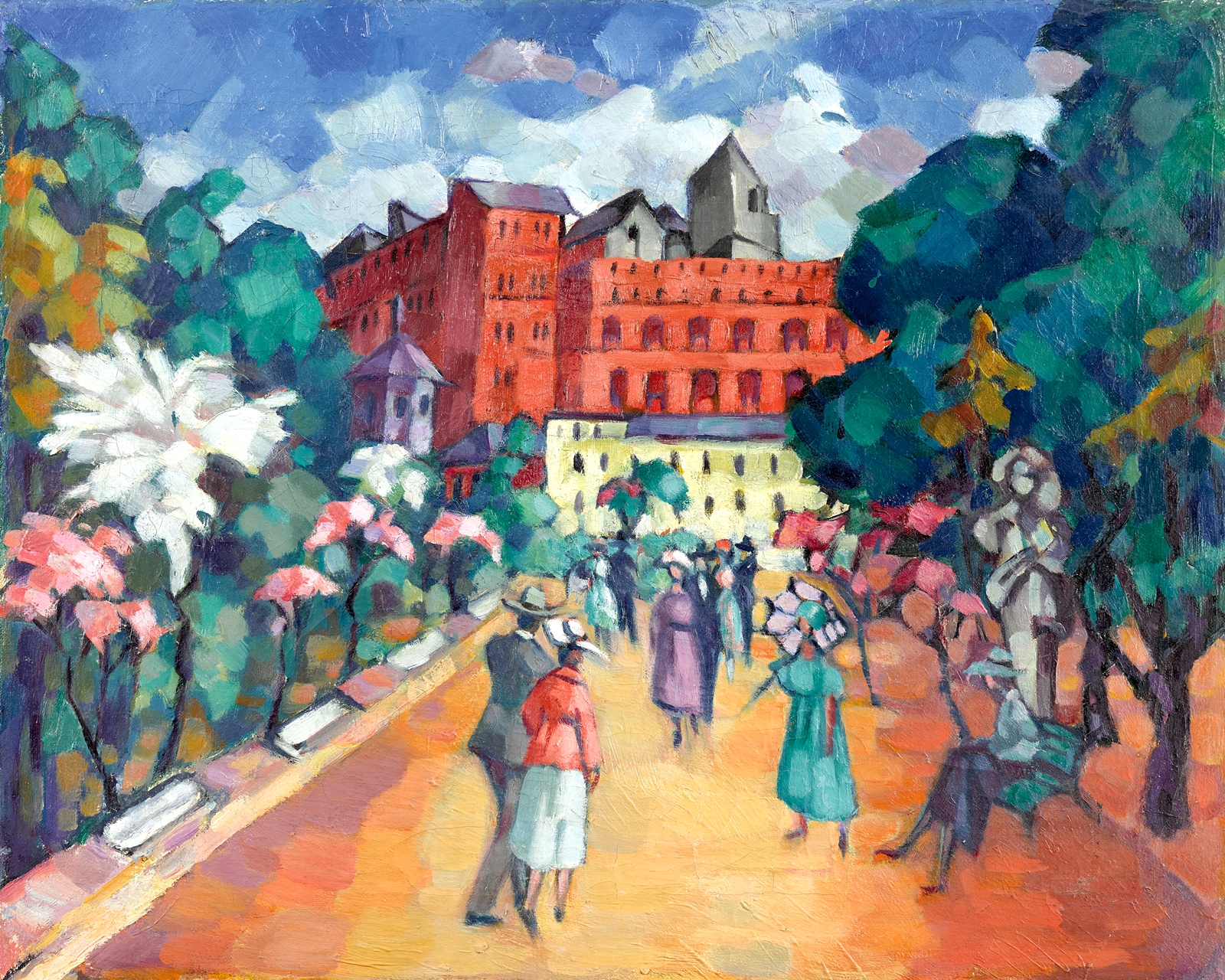The image depicts an oil painting set in a vibrant, upper-class neighborhood from the early 1800s. This impressionist-style piece features men and women in formal clothing, including men in hats and suits, and women in bonnets, umbrellas, and colorful dresses such as turquoise and lavender. The focal point is a lively street scene lined with flourishing trees and blooming pink, green, and white bushes. A woman in a bright green dress with a big hat stands prominently in the foreground, while another woman sits on a bench to the right. Further in the background stands a striking large red building with white lower facades, accompanied by smaller buildings in yellow and white. The sky is a blend of low-hanging clouds and clear blue, adding depth to the scene. A tall statue and additional distant gray buildings complete this picturesque and detailed portrayal of a bustling, elegant town center.